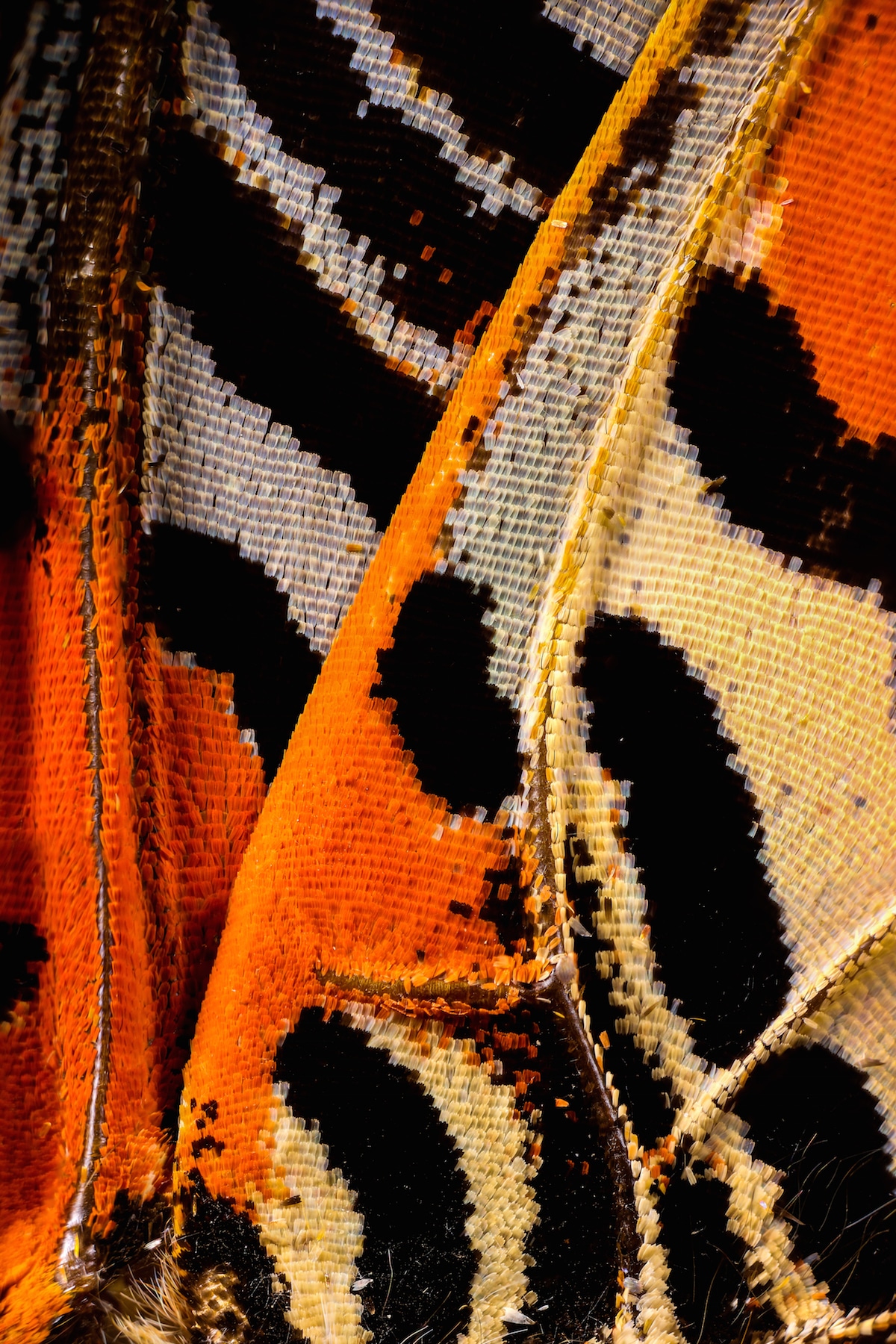The image is an extremely zoomed-in photograph of a handmade textile or artisan craft, incorporating a variety of fibers and materials. The composition includes sections of orange, black, white, beige, and pale yellow fibers, creating both striped and solid color areas. Interwoven wire can be seen running through some sections, providing structure and intricate detail. The texture and appearance vaguely resemble a butterfly wing or insect hide, with the black sections evoking the look of tiny caterpillars. At the bottom of the image, wisps of hair—potentially horsehair—are visible. The overall effect is reminiscent of a meticulously crafted rug, with vibrant colors and a sophisticated design, suggestive of a piece intended to add a pop of color and artistic flair to a living space.